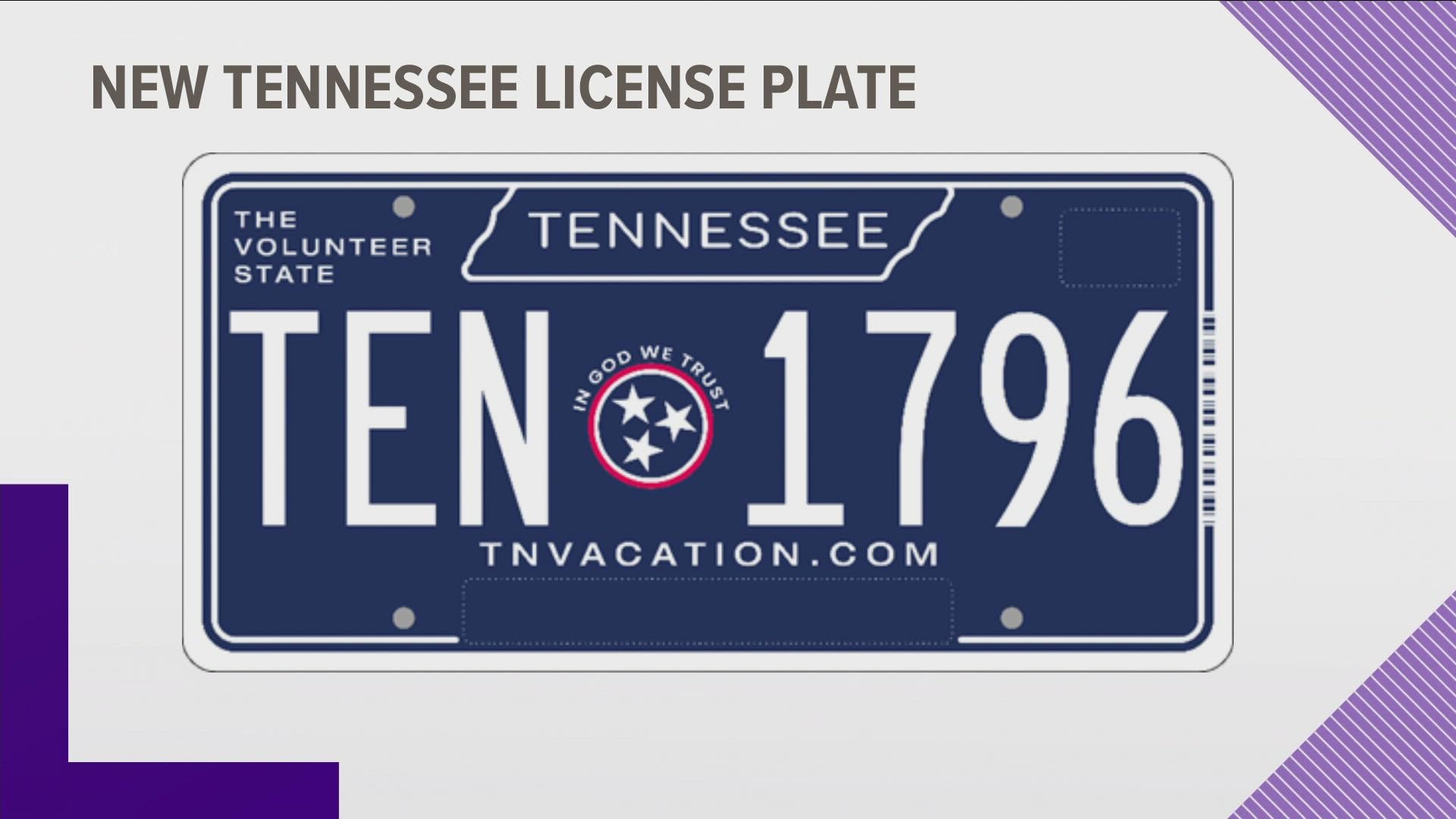This image depicts a detailed Tennessee license plate with a distinct landscape layout, where the width exceeds the height. The background primarily showcases a dark navy blue interior, contrasted by a white outer edge and multiple white lettering components. 

Across the top, in subtle gray text, it prominently reads "New Tennessee License Plate." Below, in the upper-left corner, you'll find the phrase "The Volunteer State," also in white text. Central to the plate is a significant outline of the state of Tennessee, within which the word "TENNESSEE" is boldly printed.

In large, bold lettering characteristic of license plates, the sequence "10TEN" is displayed mid-plate. A central circular emblem with a thin red outline encloses a blue center and three white stars, accompanied by the text "In God We Trust" above it in white. To the right of this, the year "1796" is presented in white font.

Additionally, the bottom edge features "TNvacation.com" in white text. On the lower left-hand corner, an L-shaped geometric symbol in dark blue, neighbored by the upper and lower right-hand corners which showcase purple triangles filled with intricate white lines, add to the plate’s distinctiveness. The collective emphasis on these repeated elements forms a comprehensive and detailed portrayal of the Tennessee license plate.